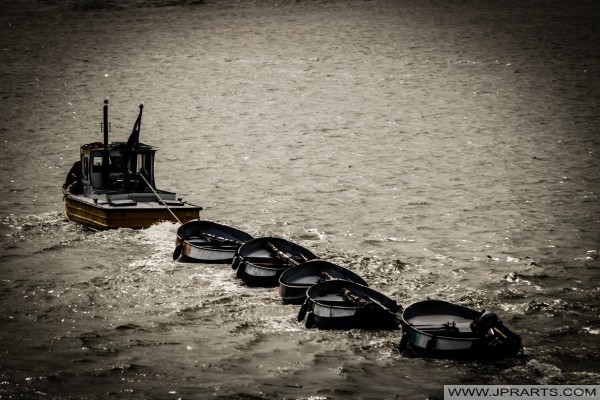The photograph, characterized by its dark lighting, captures a white and brown tugboat in open waters—possibly a bay, ocean, or large lake. The tugboat is towing five smaller boats, arranged in a line. The boats trailing appear similar in shape and are predominantly white with black bottoms; the last boat in the line clearly has a motor attached to it. There are small waves creating a rippling effect across the water, which appears to have a brownish tint, although it is unclear if this is due to a filter. The image is completely devoid of any land, trees, or other ships, providing an isolated view of the vessels. The corners of the photo are heavily vignetted, and in the bottom right corner, it prominently displays the text "www.jprts.com" within a gray rectangular box.